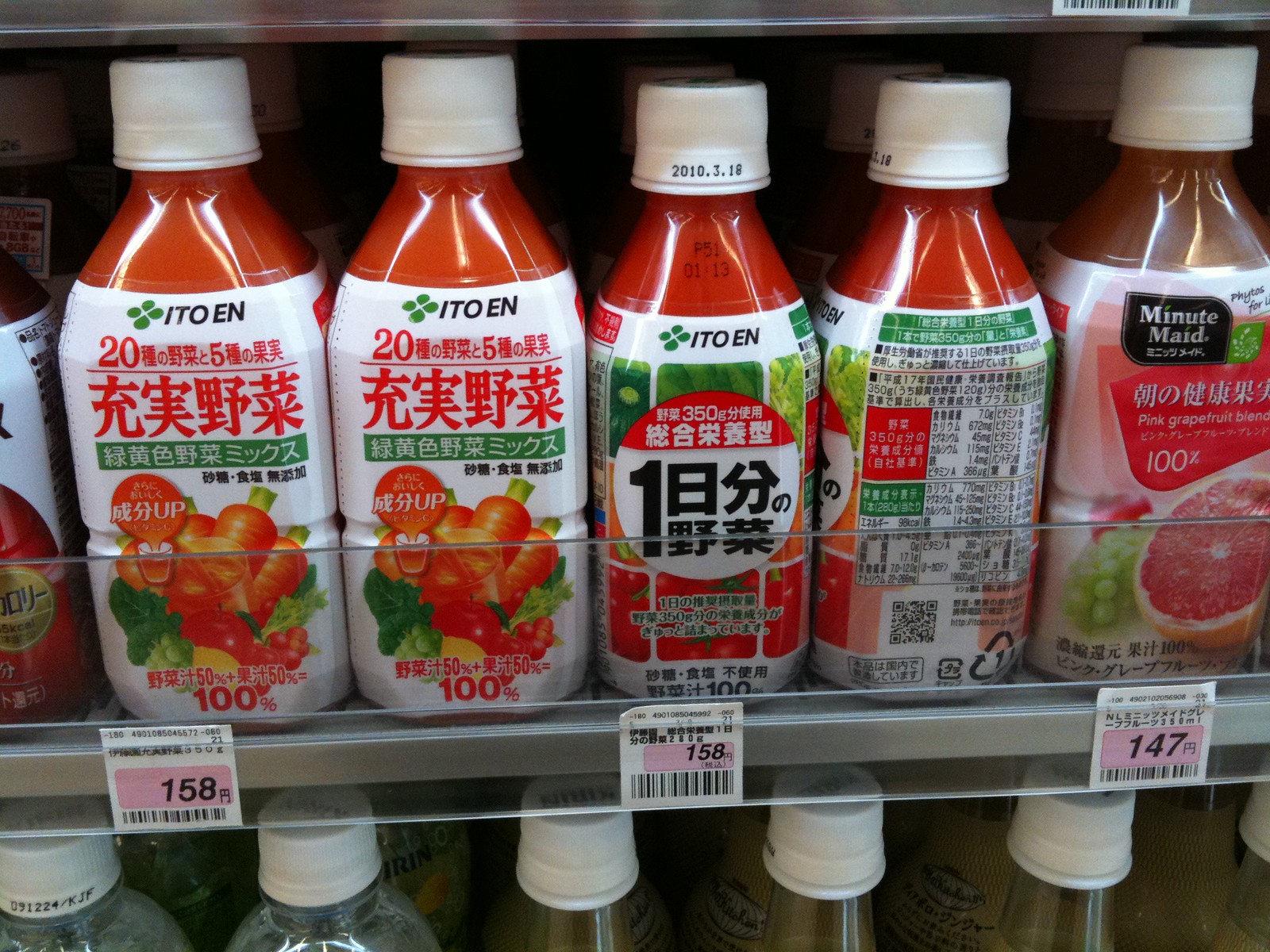The image depicts a close-up of a grocery store shelf lined with various bottled beverages, most likely of Japanese origin. The top of the shelf is grey, and part of a barcode can be seen on the right-hand side. Going from left to right, the first bottle visible has a partially obscured white label with a gold circle design. Next to it, a bottle with a white cap contains a red liquid and features a white label. This label has four dots forming a flower pattern at the top, the text "I-T-O-E-N" in black, the number "20" in red, and additional Asian characters. Beneath these, a green rectangle with more Asian characters and an image of vegetables is visible, concluding with "100%."

Continuing right, the following bottle looks similar to the previous one but has a slightly different design with an additional red circle at the top filled with Asian script. The bottle next to this appears smaller and also has a white cap and red liquid. Its label shares a similar pattern with the "I-T-O-E-N" text and a combination of red and green design elements. There's another similar bottle showing more health or nutritional information, although it's turned around and partially blurry, making the text unreadable. Its label features black and white elements, a recycle symbol, and a QR code.

Further right is a distinct bottle with a white cap and an orangey liquid labeled "Minute Maid" at the top in a uniquely shaped black rectangle. Below this are green and red design elements, Asian characters, and the words "Pink Grapefruit Blend" along with an image of a grapefruit and grapes. Price tags are visible below these bottles, reading $158 and $147, although the currency is not USD. The tops of additional bottles are partially visible beneath, indicating more products on the shelf.